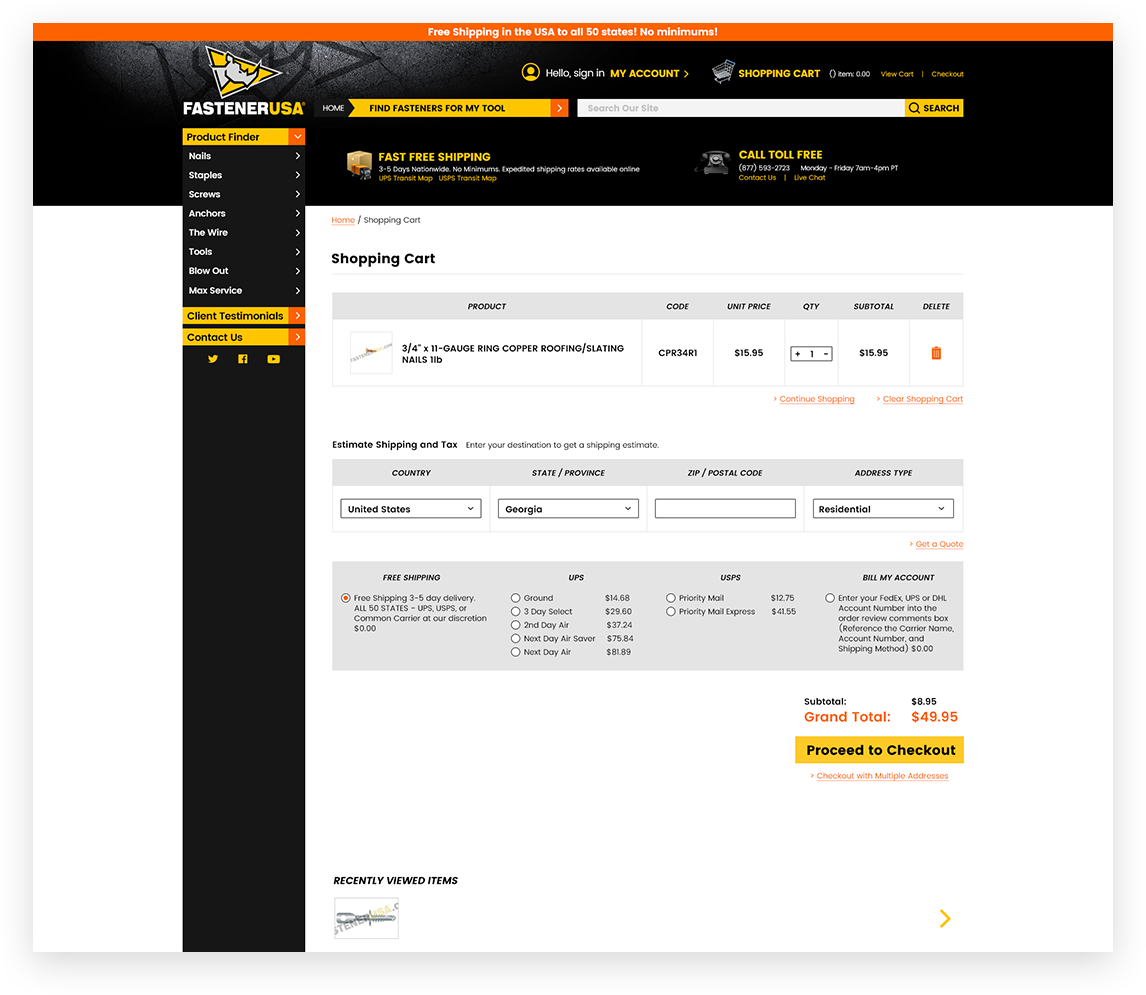**Detailed Screenshot Caption of FastenerUSA Website**

The screenshot captures the FastenerUSA website, as viewed on a computer screen. In the upper left corner, the website features a charming rhino mascot, representing the brand. Progressing towards the right, the top center of the page displays user account options: "Hello, Sign In My Account," along with the shopping cart status indicating “No items,” and options to “View Cart” and “Checkout.”

Below these options, a prominent bar reads “Find Fasteners for My Tool,” accompanied by a search bar and a search button to assist users in locating specific products. Immediately beneath this is the "Product Finder," a dropdown menu that facilitates navigation through various product categories including Nails, Staples, Screws, Anchors, Wire, Tools, Blowout, Max Service, Client Testimonials, and Contact Us. This menu is neatly arranged along the left-hand side of the screen.

At the bottom of the vertical menu, social media icons provide links to FastenerUSA's Twitter, Facebook, and YouTube pages.

To the right of the menu, the main shopping cart section displays a detailed view of a selected product: "3/4 inch 11 Gauge Ring Copper Roofing Nails - 1 Pound." The product code is listed, priced at $15.95 per unit with an option to delete the item. 

Further down, shipping details are outlined with options to estimate shipping and taxes based on location—specified in this instance as the United States, Georgia, and an empty postal ZIP code field. The shipping address type is categorized as residential.

At the bottom of the cart, various shipping methods and their costs are displayed: free shipping (USPS 3-5 day), Ground ($14.68), Three-Day ($29.60), Second Day Air, Next Day Air, Priority Mail ($12.75), and Priority Mail Express ($41.55). An option to “Bill My Account” is also available.

Finally, the subtotal of $8.95 escalates to a grand total of $49.95 with added shipping costs, clearly stated before the “Proceed to Checkout” button, inviting the user to complete their purchase.